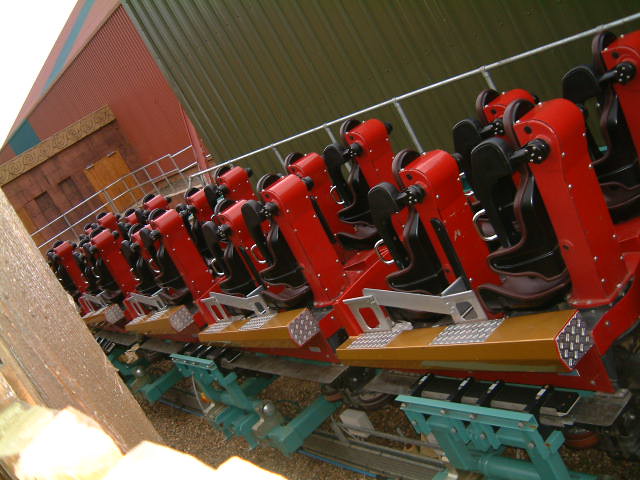The photograph depicts a detailed scene of the seating area for a roller coaster at an amusement park. The individual seats are lined up in multiple rows, accommodating three or four riders per row, with the seats designed in dark brown leather or vinyl material that ensures riders sit upright. The backs of the seats are accentuated with red metal panels, which are detailed with silver studs and appear to provide structural support to keep the seats steady. The seating unit is integrated with a rail system and is bordered by a sturdy silver metal railing. To one side of the seating area, there is a green metal wall, possibly resembling the side of a shipping container. On the opposite side, there is a steel diamond plate and a pebble-type gravel path beneath the structure. A brass or yellow platform offers a stepping area for riders to board the roller coaster, completing the elaborate setup with various elements of red, black, silver, green, and brown, contributing to the vibrant and industrial aesthetic of the scene.